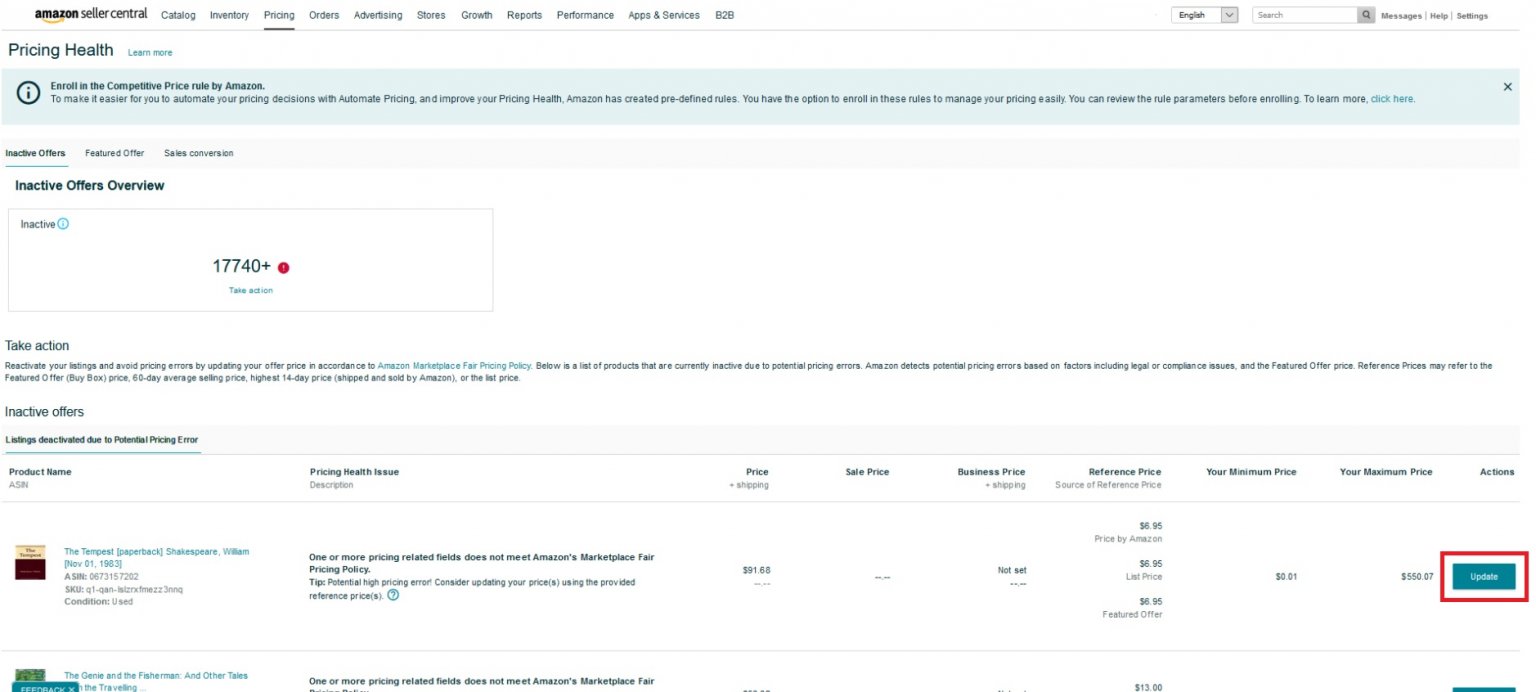Here is a cleaned-up and detailed caption for the given image description:

---

This image is a screenshot in portrait mode from Amazon Seller Central, specifically the "Pricing" page. The page has an organized layout with several tabs displayed across the top: Catalog, Inventory, Pricing (underlined), Orders, Advertising, Stores, Growth, Reports, Performance, Apps and Services, and B2B. 

At the upper right-hand corner, there are drop-down menus including language selection set to English, and options for Messages, Help, and Settings, alongside a search bar.

Below this, the page displays a section titled "Pricing Health" in bold, accompanied by a light green link labeled "Learn more." Following this, there's a green-backgrounded banner promoting the "Competitive Price Rule by Amazon," encouraging sellers to use Amazon's predefined rules to automate their pricing decisions and improve pricing health. The banner includes a blue "Click here" link for more information, and an option to close the message.

The main content area features a row with tabs for different types of offers: Inactive Offers, Featured Offers, and Sales Conversion. The "Inactive Offers" tab is selected.

Within this tab, there is a light gray-bordered content box detailing inactive offers, currently totaling 1,774 items, indicated by a red exclamation point. An alert message advises sellers to reactivate their listings and avoid pricing errors by updating their offer prices to comply with Amazon's Marketplace Fair Pricing Policy. This message is highlighted in green.

On the right-hand side, there are various selection options along with a prominently displayed green "Update" button, which is highlighted in red, indicating the urgency for action to update inactive offers.

---

This revised caption provides a clear and detailed description of the screenshot, making it easier to understand the contents and context of the image.